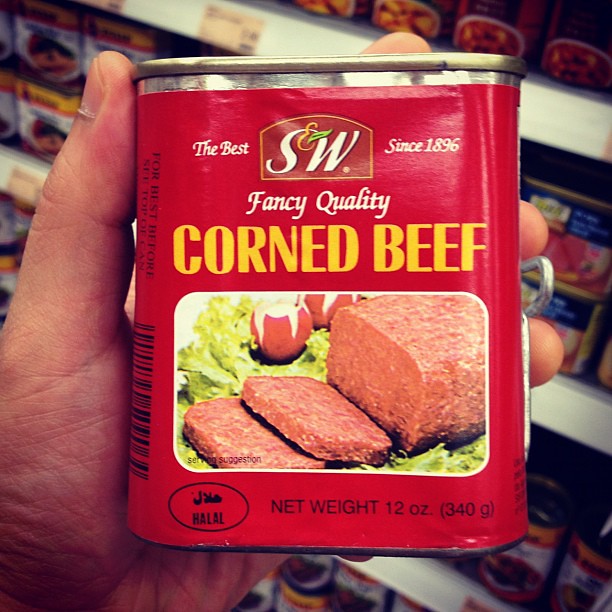In the image, a fair-skinned individual is holding a can of premium-quality corned beef. This square can, bearing the brand S&W, has the company's logo and the tagline "The Best" prominently displayed at the top, and it states that the brand has been established since 1896. The can weighs 12 ounces or 340 grams. Notably, in the bottom left-hand corner of the can, there is an oval emblem resembling an egg shape with "Halal" inscribed inside, indicating that the product meets Halal dietary standards. In the background, the scene appears to be a store aisle with shelves stocked with a variety of canned goods. Among these items, several other cans of the same corned beef are visible, alongside an assortment of blue and round cans, suggesting a well-stocked grocery environment.